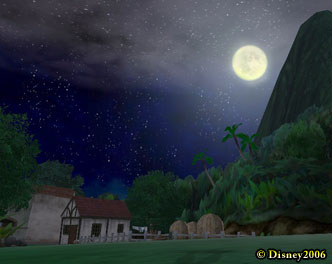This detailed painting, reminiscent of a video game scene, depicts a serene nighttime landscape under a starlit sky. Dominating the upper right portion of the canvas, a glowing full moon peeks through thin, misty clouds, casting a soft light over the scene. To its right, a smooth-edged, grayish mountain rises majestically, its base surrounded by lush green trees. The foreground features a vibrant green grassy field, dotted with neatly stacked bales of hay toward the right. On the bottom left, a prominent yellow logo reads "Disney 2006," denoting the artwork's origin. Two charming cottages occupy the left side: one is white with brown trim, a red roof, three windows, and a door, while the second structure, visible from the side, also sports a red roof. The tranquil night sky, spanning across the painting, is a rich dark blue filled with countless stars, enhancing the dreamlike quality of this idyllic scene.